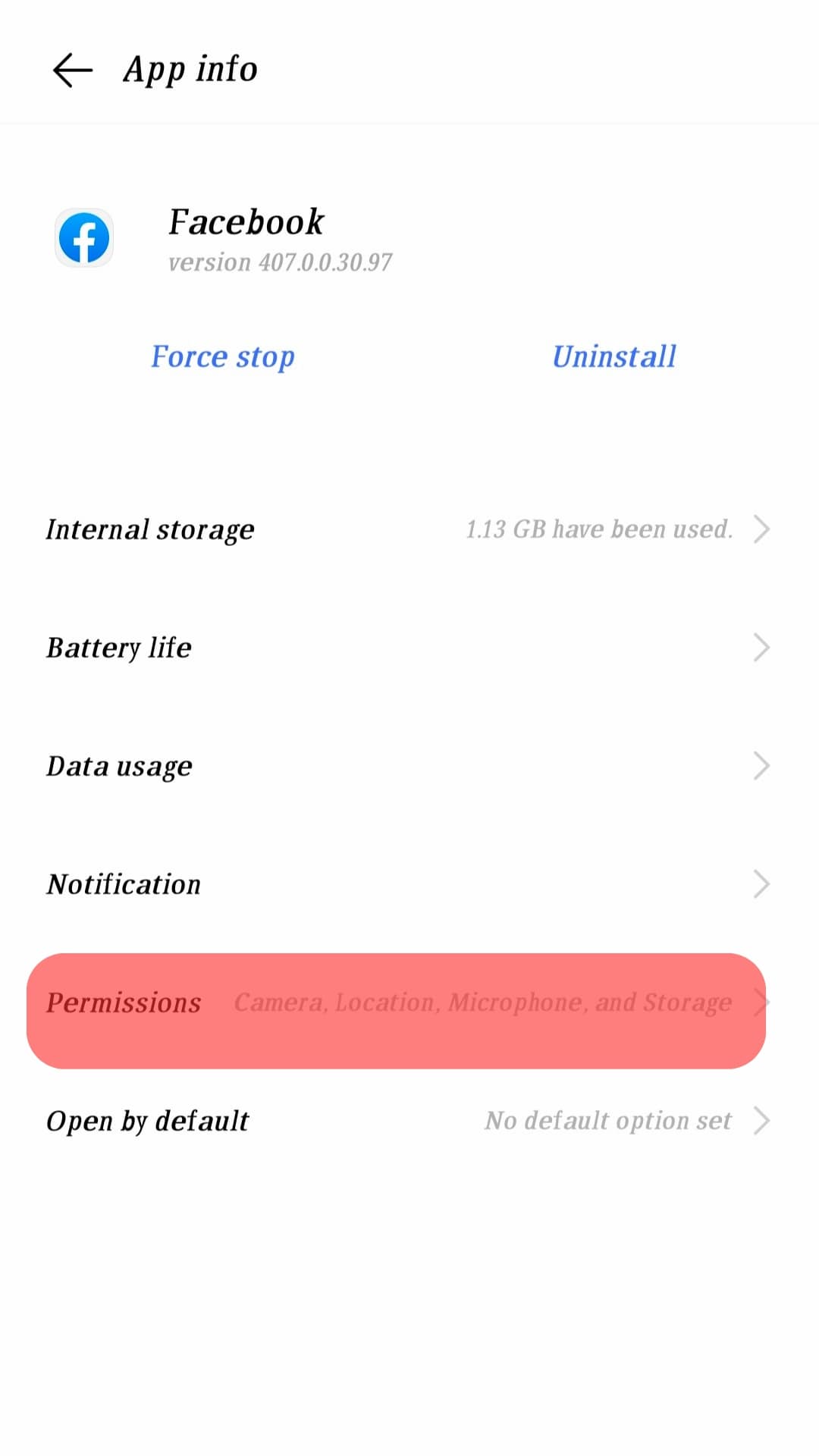The image appears to be a screenshot taken from a cell phone, showing the "App Info" page for the Facebook application. The background is white. 

At the top left corner, there are black letters reading "App Info" with a left-pointing arrow preceding the text. Directly under this heading, it says "Facebook" in black font, followed by "version 4.0" in black and underneath that, a gray text version "407.0.0.30.97". To the left of the "Facebook" text, there is a blue circle containing the Facebook icon.

Beneath the version information, there is a blue button labeled "Force Stop" on the left and "Uninstall" in blue text on the right.

Further down, the text "Internal storage" is displayed in black, and to the right of this, in light gray text, it states "1.13 GB used" with an arrow pointing to the right.

Following this are the sections labeled "Battery," "Data usage," and "Notifications," each presumably with further details that are not visible in the image.

In a red rectangular area with rounded corners (darker red on the left), it says "Permissions" in a dark red font, and next to this in a lighter red color, it lists "Camera, Location, Microphone, Storage."

Below, to the left, it says "Open by default" in black. To the right of this, in gray text, it states "No default options set."